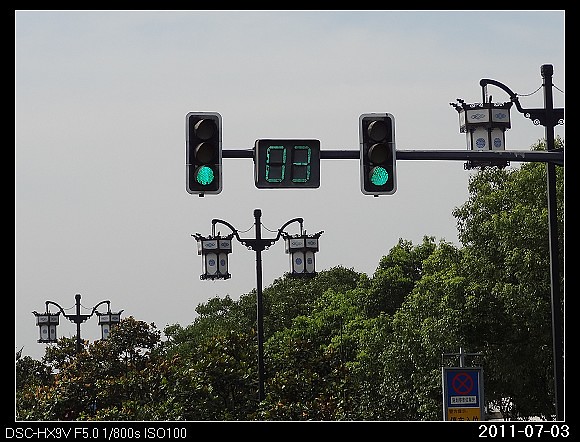The image portrays a modern traffic light setup, likely from an Asian country due to the intricate lantern-like lamps with blue and white designs resembling Asian calligraphy. In the foreground, two green traffic lights indicate 'go,' while centrally positioned between them, a digital display shows the number '03,' suggesting a countdown system. The scene is enhanced by several posts adorned with black lanterns featuring these detailed patterns. Beyond the setup, a lush backdrop of trees and an open sky create a serene environment. The photo, dated July 3rd, 2011, appears to have been taken with a high-quality camera, as indicated by the label "DSC-HX9B."